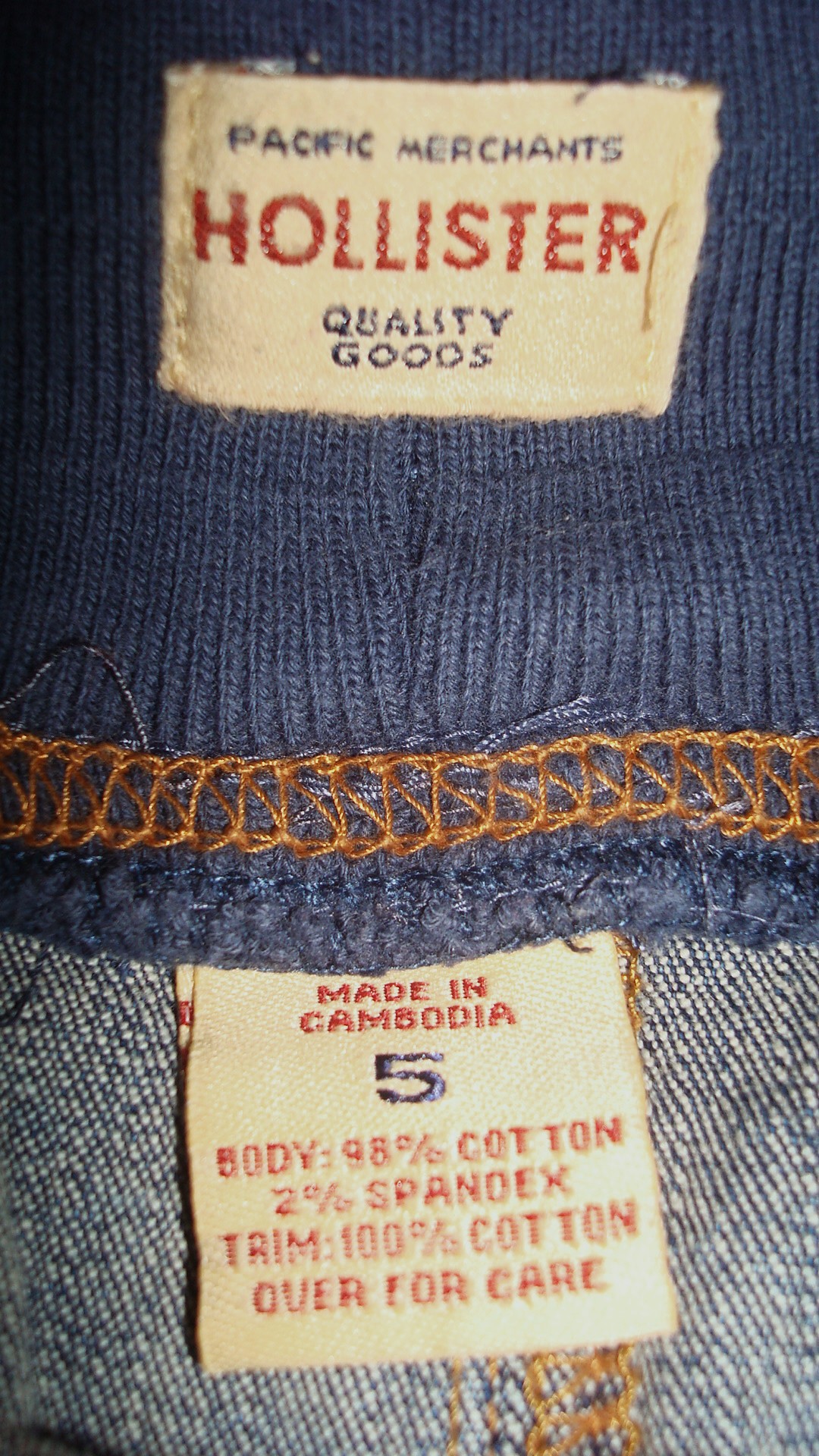This image features a blue jean garment prominently displayed. The lower section of the garment showcases classic blue denim material accentuated by contrasting golden stitches. The attention to detail is evident in the craftsmanship of these stitches. Attached to this section is a white square tag with the following details: "Made in Cambodia" written in red, "Five Below" written in blue underneath, and further down in red, it reads "Body: 98% Cotton, 2% Spandex, Trim: 100% Cotton." Below these details, it advises to "Turn Garment Inside Out For Care Instructions."

The upper portion of the garment is made from a darker blue material, creating a visually appealing two-tone effect. Affixed to this section is another white rectangular tag bearing the brand name "Pacific Merchants" in a distinguished script. Directly beneath the brand name, "Hollister" is written in red, and under that, "Quality Goods" is inscribed in blue. The tags and stitching collectively offer a glimpse into the garment's origin, material composition, and brand identity.